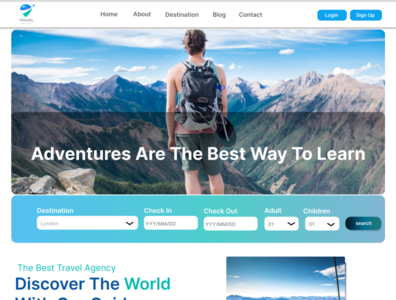The image depicts a webpage captured in low quality, appearing blurry, fuzzy, and somewhat pixelated. The text within the image is small and unclear due to the diminished resolution. In the top right corner, there are two distinct buttons: one labeled "Login" and the other "Sign Up." Centrally aligned at the top of the page are five navigation tabs labeled, from left to right, "Home," "About," "Destination," "Blog," and "Contact." On the top left, there is a small, indistinguishable icon featuring blue and green colors.

Positioned prominently in the middle of the webpage is the text "Adventures are the best way to learn." The background showcases the back view of a person with brown hair, who is wearing a tank top, a green backpack, and green shorts.